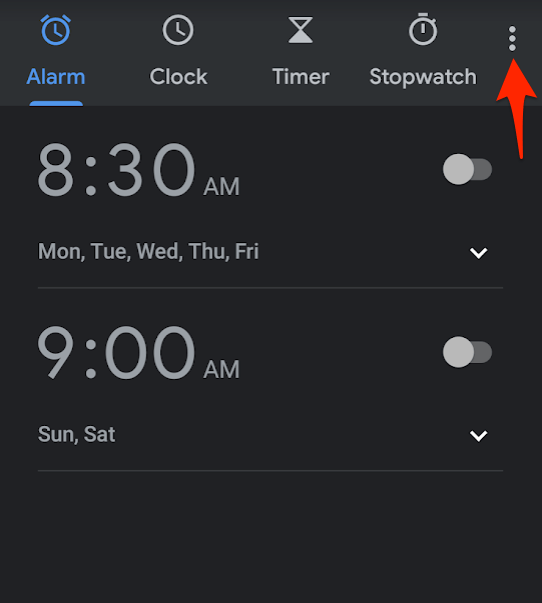This image appears to be a screenshot taken from a mobile webpage or application, displaying the interface of a clock app. The background is predominantly black, contributing to a sleek and modern design. At the top of the screen, there are four options: "Alarm," which is highlighted in blue with an underline indicating it has been selected, "Clock," labeled in white with a white clock icon above it, "Timer," represented by an hourglass icon with filled lower triangle, and "Stopwatch," accompanied by a stopwatch icon.

A prominent red arrow draws attention to three vertically aligned dots located on the right-hand side, likely indicating a menu or additional options. Below this, the screen shows two alarm settings: one for 8:30 a.m. from Monday to Wednesday and Thursday to Friday, which is currently turned off, and another for 9:00 a.m. on Sunday and Saturday, also turned off, as indicated by the position of their respective sliders.